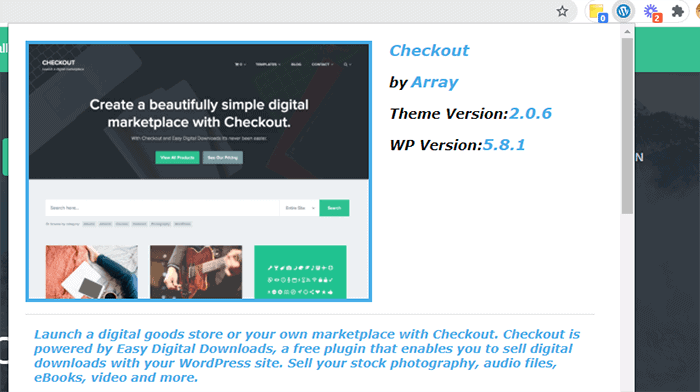A website interface is displayed, dominated by a prominent box that reads "Check Out Here" in white text, although it is somewhat difficult to discern. Below this box, an expandable series of options is presented, featuring individual drop-down menus for various categories that are also not easy to read. The primary slogan, "Create a beautifully simple digital marketplace with Checkout," is prominently displayed in larger, readable font across two lines.

Subsequently, additional explanatory text elaborates on the benefits of the Checkout feature and the convenience of easy digital downloads. A green button labeled "View All Products" and another one that says "See Our Pricing" in white text against a gray background are situated below. A search bar labeled "Search Here" is also available, accompanied by a drop-down menu currently set to "Entire Site," and a green "Search" button adjacent to it.

Further down, there is a visual section with three images: one depicting a woman sitting on a bed with a tablet and notepad, clad in jeans without socks but only her pant leg visible; another of a man playing a guitar using a pick; and a third image that appears to showcase hieroglyphics or keyboard symbols.

At the bottom section in blue, the text encourages users to "Launch a digital goods store or your own marketplace with Checkout." It emphasizes that Checkout is powered by "Easy Digital Downloads," a free plugin that allows users to sell digital products on their WordPress sites, including stock photography, audio files, ebooks, videos, and more. Across from this message, the site version information is displayed: "Create a Beautifully Simple Digital Marketplace - Checkout by Array Theme Version 2.0.6" and "WP Version 5.8.1."